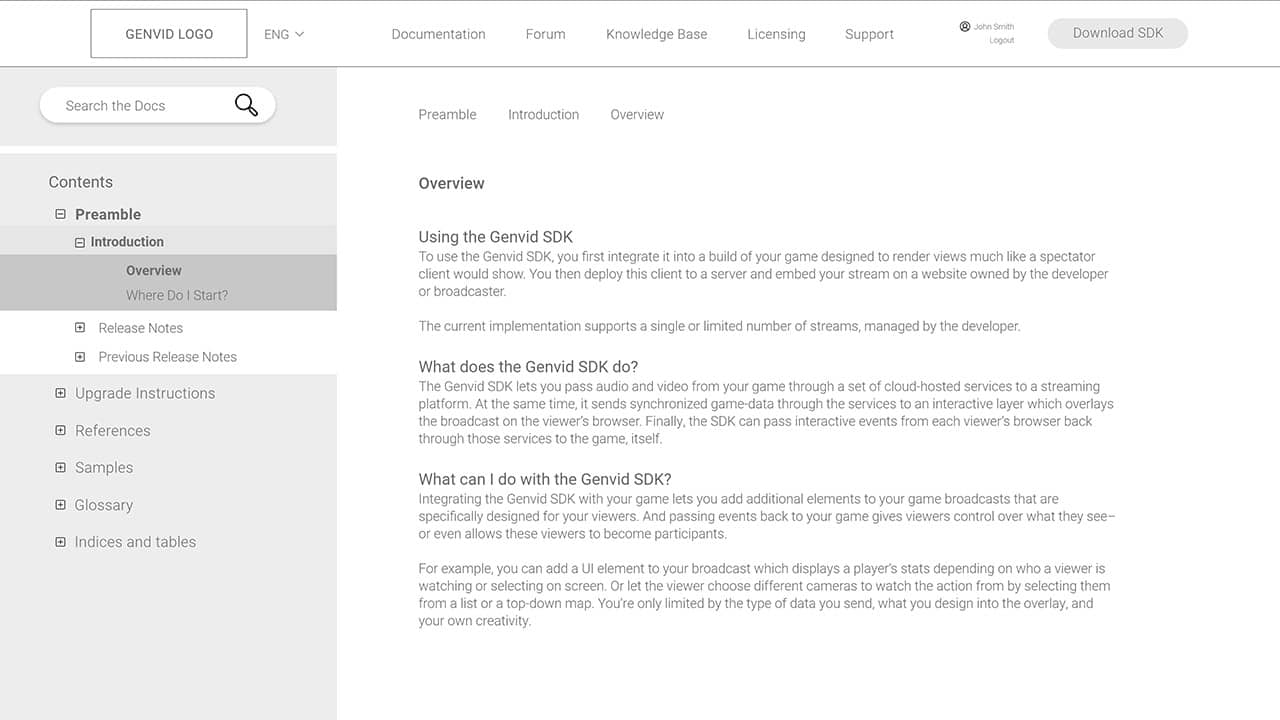The image depicts a webpage with a predominantly white background and a gray header section. The gray lines in the header section demarcate various elements. The top left corner features the GenVid logo, followed by the text "Eng" indicating the language option, English. Adjacent to these elements, a navigation menu includes links labeled "Documentation," "Forum," "Knowledge Base," "Licensing," and "Support," each separated by a small space.

On the right side of the header, there is a circular icon with the name "John Smith" next to it, accompanied by a "Log Out" option and a "Download SDK" button.

On the left sidebar, several sections are listed under a search bar labeled "Search the Docs." These sections include "Contents," "Preamble," "Introduction," and an "Overview" highlighted in a darker gray rectangle with the text "Where Do I Start." Beneath this, within a white rectangle, are links to "Release Notes" and "Previous Release Notes."

Further down, in a light gray area, there are additional sections: "Upgrade Instructions," "References," "Samples," "Glossary," "Indices," and "Tables." Each section is followed by a checkbox icon with a plus sign.

The central part of the image, presumably the main content area, contains an overview section featuring questions and answers, providing further details and guidance on the website's offerings.